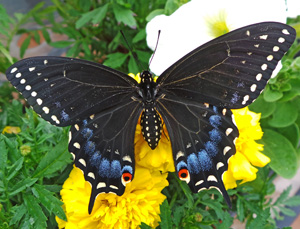An outdoor close-up image features a striking butterfly perched delicately on a yellow flower, which appears to be a vibrant marigold. The butterfly is the focal point of the photograph, boasting a stunning color palette with its upper wings displaying a deep blue-black hue. The lower halves of its wings transition to a lighter shade of blue, with a distinct band of even lighter blue following the edge of the darker region. A row of white spots adorns the very edges of the wings, continuing around the bottom halves, enhancing the butterfly's intricate beauty. The butterfly’s body is black, complemented by two prominent antennae. The background offers a lush backdrop of green leaves, reminiscent of rose foliage, creating a natural and serene setting for this captivating moment in nature.